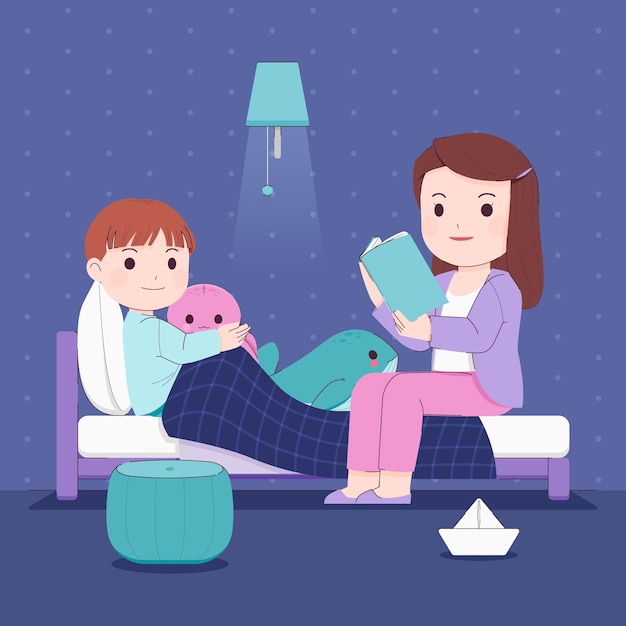The image portrays a digital cartoon scene featuring a mother reading a bedtime story to her son in a highly stylized, predominantly purple room. The background is defined by purple walls adorned with white polka dots and a turquoise lamp fixed above, casting a blue-green light. The floor is deep purple, adding to the room's whimsical ambiance. The boy lies at the head of a purple bed with a white mattress and a dark blue blanket covering his feet. He wears light blue pajamas and has a simple, expressive face with two black dot eyes, a small line for a smile, and two blush stickers on his cheeks. His reddish-brown hair is cut in a bowl style. He clutches a stuffed pig and is accompanied by other plush toys, including a mint-colored whale and a pink octopus. 

At the foot of the bed sits the mother, a woman with long brown hair stretching past her shoulders. She wears a purple jacket over a white shirt, pink pants, and matching purple slippers. The mother has a more detailed cartoon face with red lipstick and a gentle smile. She reads from an open turquoise book, indicating an engaging storytelling moment. In the room's foreground, a turquoise seat cushion and a paper boat add to the playful decor. The overall scene exudes a cozy, intimate bedtime routine set in a vividly colored, child-friendly environment.